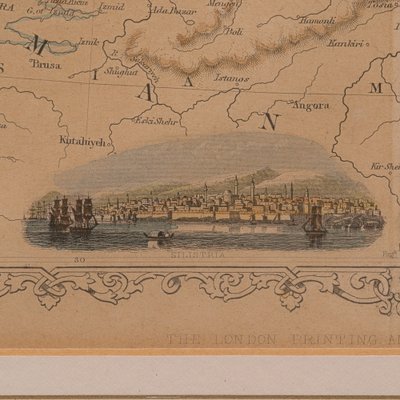The image is an old-style map depicting various regions with black outlines and names such as Angora, Cuta de Lea, and Prusa sketched at the top. Below these outlines, there is an intricate inset of a picturesque port town situated by a river or perhaps a harbor. The town features numerous spires and towers, with smaller buildings nestled below and a backdrop of brown, snow-capped mountains. In the water, which is shaded blue like the sky, three brown sailing ships are visible: two on the left with multiple levels of sails sailing toward the city, and one on the right with a single layer of sails going leftward. Additionally, there's a smaller boat in the center. The harbor scene is complemented by elements like tall smokestacks and coal-burning factories. The lower third of the image showcases a decorative border featuring black spirals on a beige background, with some text that is hard to read, and a distinctive bottom border in white. The bottom also includes a mention of "The London Printing," adding to the old-fashioned charm of the piece.